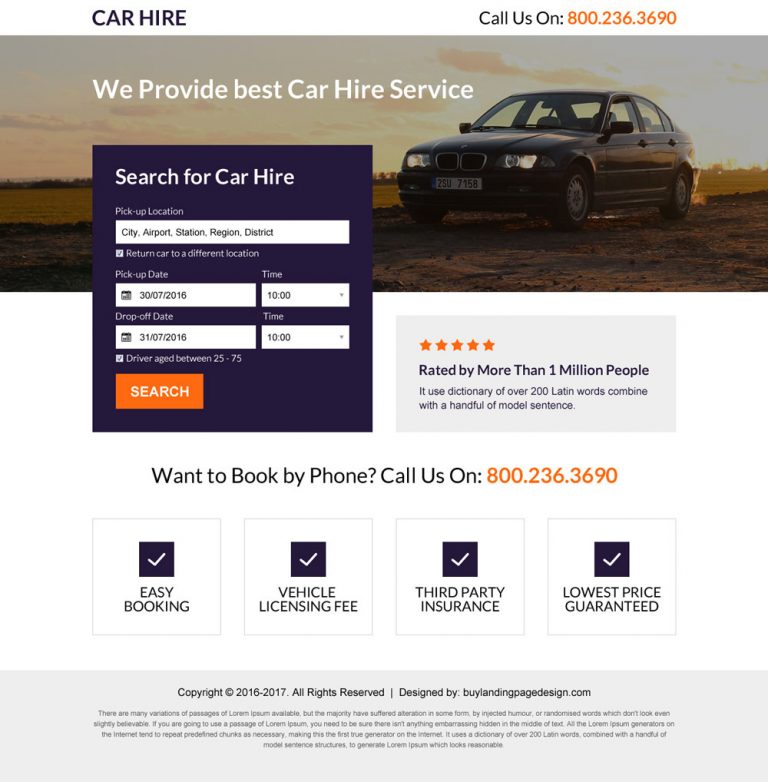**Detailed Caption:**

The image features a car hire advertisement with various elements and details:

- **Top Left**: The text "Car Hire" is displayed in purple.
- **Top Right**: An orange-colored contact number, "Call us on 800-236-3690". Below it, the phrase "We provide the best car hire service" is written in white text.
- **Main Background**: The background features a navy BMW car facing left. The ground is brown, and the sky behind the car is yellow with some clouds.
- **Left Tab**: There is a purple tab on the left side with several fields and options for searching car hires:
  - A white square with purple text that reads "Search for car hire".
  - Categories for picking a location: "City, Airport, Station, Region, or District".
  - An option to return the car to a different location, with a checked checkbox.
  - Fields for entering pick-up and drop-off dates and times.
  - A checked checkbox for the driver age requirement "between 25 to 75".
  - An orange "Search" button.
- **Right Section**:
  - The rating "5 star rated" is displayed with yellow stars and purple text.
  - A statement reads: "Rated by more than 1 million people".
  - A note about using a dictionary with over 200 Latin words combined with model sentences.
  - Contact information: "Want to book by phone? Call us on 800-236-3690".
- **Bottom Section**:
  - There are three purple squares with white text and checkboxes:
    - Left: "Booking is easy".
    - Middle: "Vehicle licensing fee".
    - Right: "Third-party insurance".
  - A statement ensuring "Lowest price guaranteed".
  - A footer with blurred text in black that includes "© 2016-2017 All rights reserved" and a note about the design, "Designed by LandingPagesDesign.com".

This advertisement effectively highlights key details and offers for potential car hire customers.